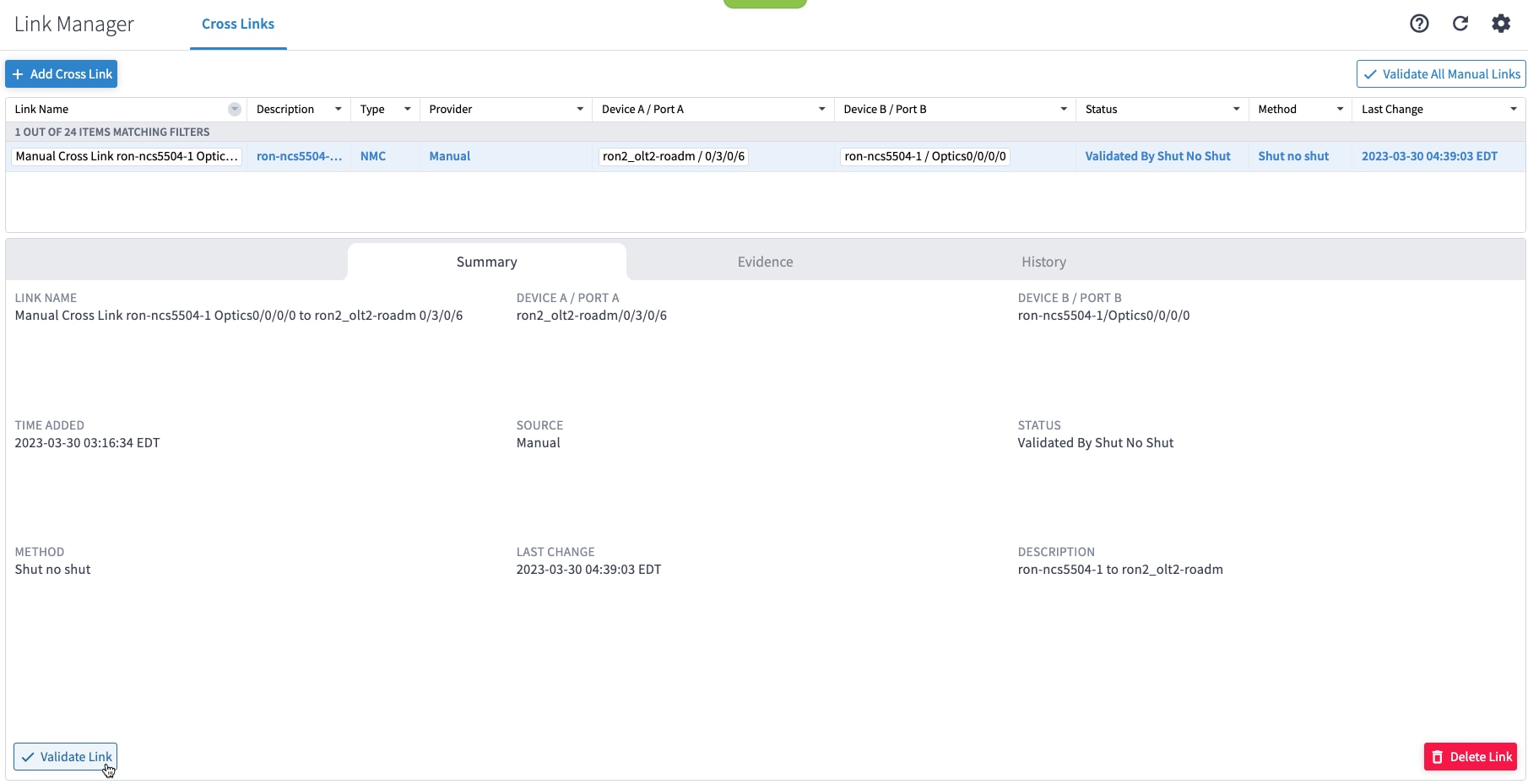This is a detailed digital screenshot displaying various items related to the manual crosslink of the RON-NCS5504-1 optic. The summary section provides an overview of the process. Additionally, the timestamp indicates when the items were added, and the status shows that validation was performed by SHUT, although no issues were flagged during this process. There is also an option to access the validation link for further details.